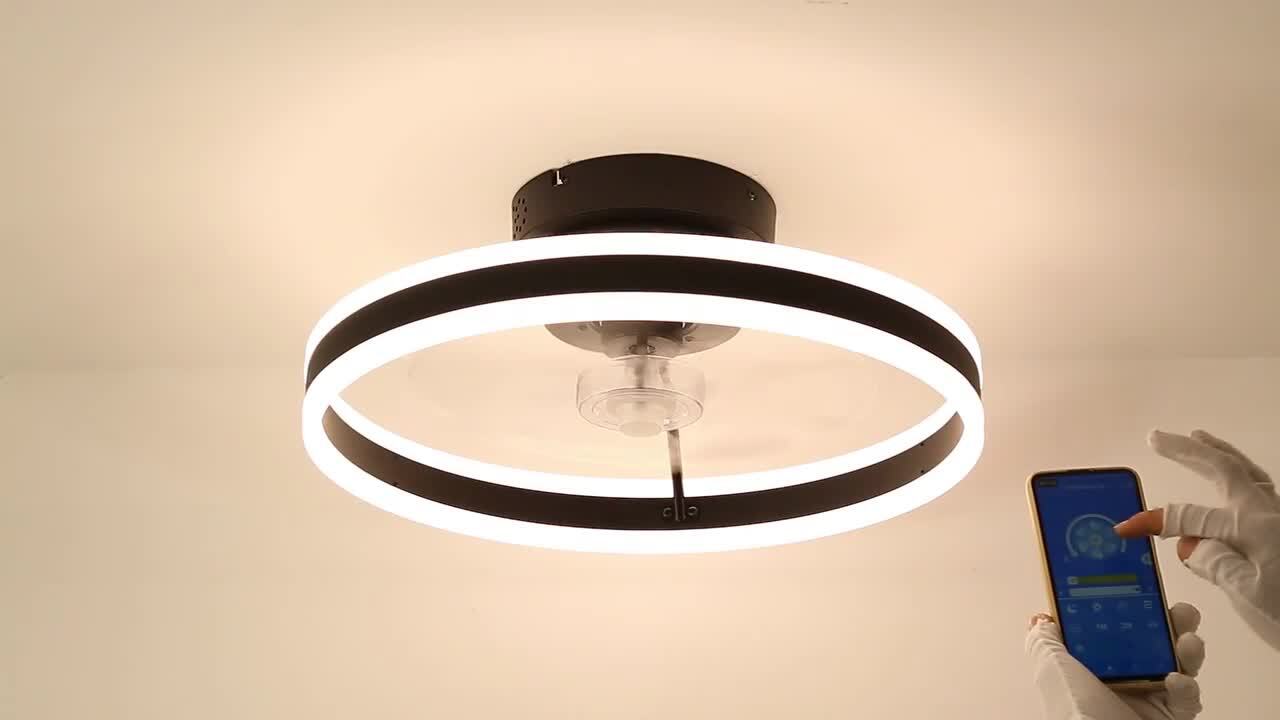This detailed close-up photograph captures a sophisticated modern ceiling light fixture with a round, black base securely mounted to a light cream, slightly rose-tinged ceiling. Extending from the base is a cylindrical light element featuring a distinct black stripe that wraps around its midsection, dividing it into two luminous sections that emit light both upwards and downwards. Intriguingly, the center of the base has a small, silver, round component, potentially indicating a concealed fan mechanism. In the lower right corner, an adult's hands, partially wrapped in gauze-like white gloves with the index and thumb fingers cut out, are visible. These hands hold and interact with a smartphone displaying a dark blue screen, seemingly using an app to program or control the ceiling light. The glimpse of the partial white wall next to the ceiling completes the ambient setting of the room.